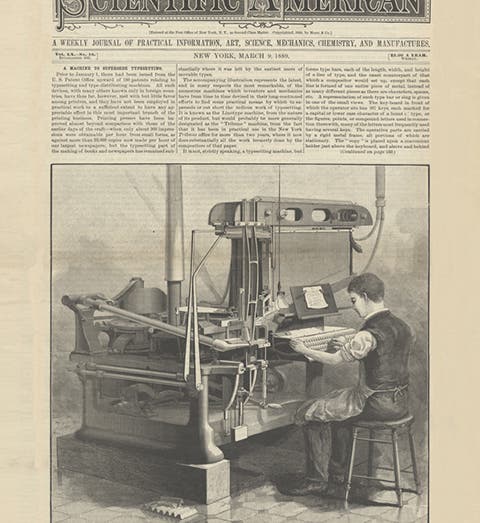The vintage black and white print piece, vertically rectangular in shape, depicts a detailed scene dominated by a Caucasian male with short hair, sitting on a stool. He is dressed in a dark shirt and pants, covered by a white apron. Occupying most of the bottom two-thirds of the image, the man is intently working on an old-style printing press, likely setting up typeset tiles. The image is framed by a thin black border and placed against a light brown background.

At the top of the image, there's a partially cut-off banner, suggesting it might say "Scientific American." Below the banner, in smaller, readable print, it states: "A Weekly Journal of Practical Information, Art, Science, Mechanics, Chemistry, and Manufacturers. New York, March 9th, 1888." This detailed and highly illustrative piece exudes historical charm and captures a moment of industrious activity, emphasizing its focus on the era's technological and industrial advancements.